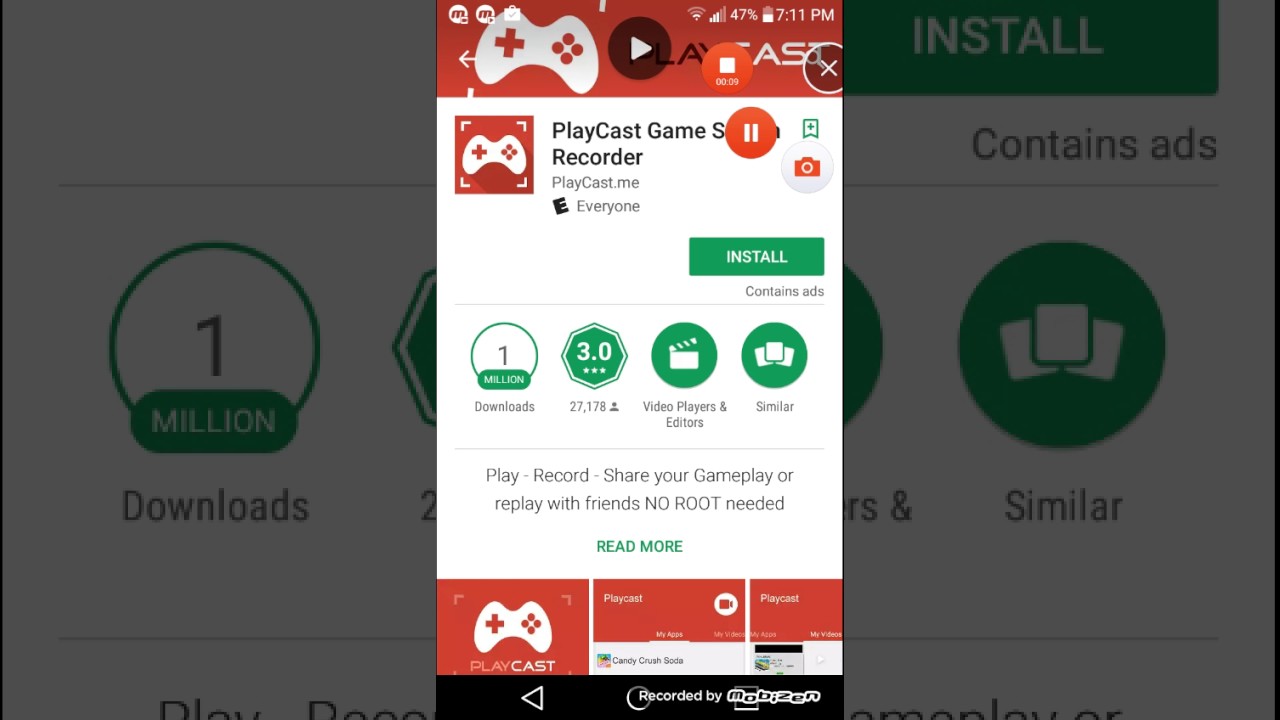The image showcases a detailed pop-up window superimposed on a gray-out website, preventing any interaction with the background elements. The pop-up, which is predominantly white and accentuated with red and green graphics, is an advertisement for a gaming application. 

At the top, it is labeled "Playcast Game Recorder," though the word following "Playcast Game" is partially obscured by a pause button. The left side features a game controller icon next to the tagline "Cast Me." The game boasts an E for Everyone rating, includes a camera icon supposedly to display game snapshots, and highlights a green "Install" button, indicating that the game contains ads.

Below this, there are indicators of the game's popularity, such as "1 million downloads" and a "3-star rating" from 27,178 reviews. Additionally, the pop-up categorizes the app under "Video Players and Editors" and suggests "Similar" applications. A horizontal separator divides this information from the promotional tagline: "Play, Record, Share Your Gameplay or Replay with Friends, No Root Needed," accompanied by a "Read more" link.

At the very bottom, the pop-up showcases several graphics: a clear depiction of a controller labeled "Playcast," another showing "Playcast and Candy Crush Game," and a third blurred image. The final text mentions that the recording functionality is provided by "Mobizen."